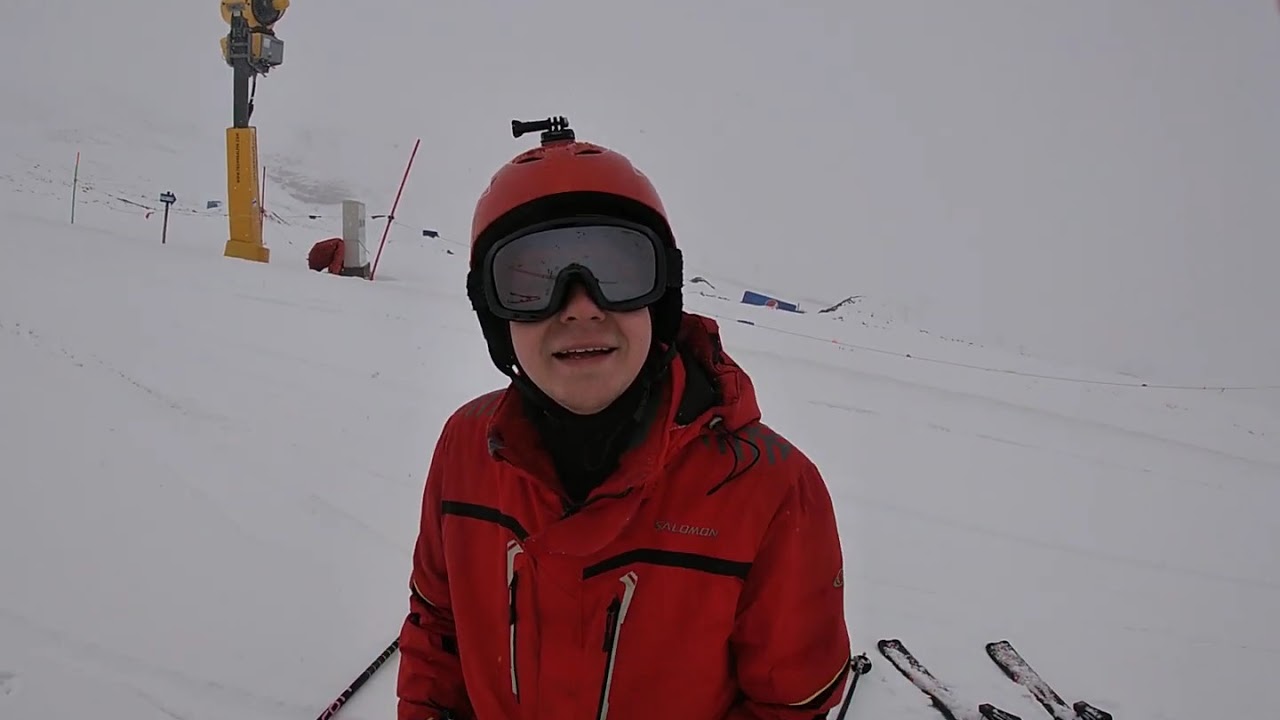The image captures a skier, possibly a young boy, standing in the center of a snowy ski slope. He is wearing a bright red jacket with black stripes and multiple zippers. His hood is down and on his head is a red and black helmet equipped with a mount for a camera, though no camera is attached. He has black-rimmed ski goggles on and is smiling. To the lower right of the image, the tips of skis are visible on the snow. Behind him, the slope descends from left to right, featuring a large pillar with yellow padding at the base and dark gray metal at the top. Various square-shaped lights are mounted on this pillar. In the distance, thin poles with lines of triangle-shaped flags are seen against a dark gray sky, adding to the wintery atmosphere.